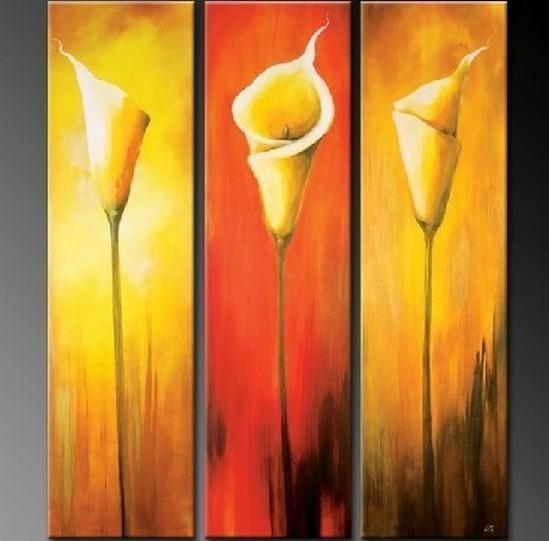This image displays a striking triptych of floral portraits. Each of the three vertical paintings features a single long-stemmed flower with a distinctive bowl-shaped bloom, possibly lilies. The flowers themselves are primarily yellow and white, with subtle hints of orange. The left panel has a yellow background that blends into a reddish-orange at the bottom, with the flower facing to the right. The middle panel features a dark red background with the flower facing forward, showcasing the full cup of the bloom. The right panel has a yellow background that transitions into gray at the bottom, with the flower facing to the left. All backgrounds are artistically blurry blends of colors, enhancing the realism of the flowers. These paintings are mounted on a wall that transitions from a lighter gray on the left to a darker, almost black hue on the right, creating a cohesive and visually appealing display.